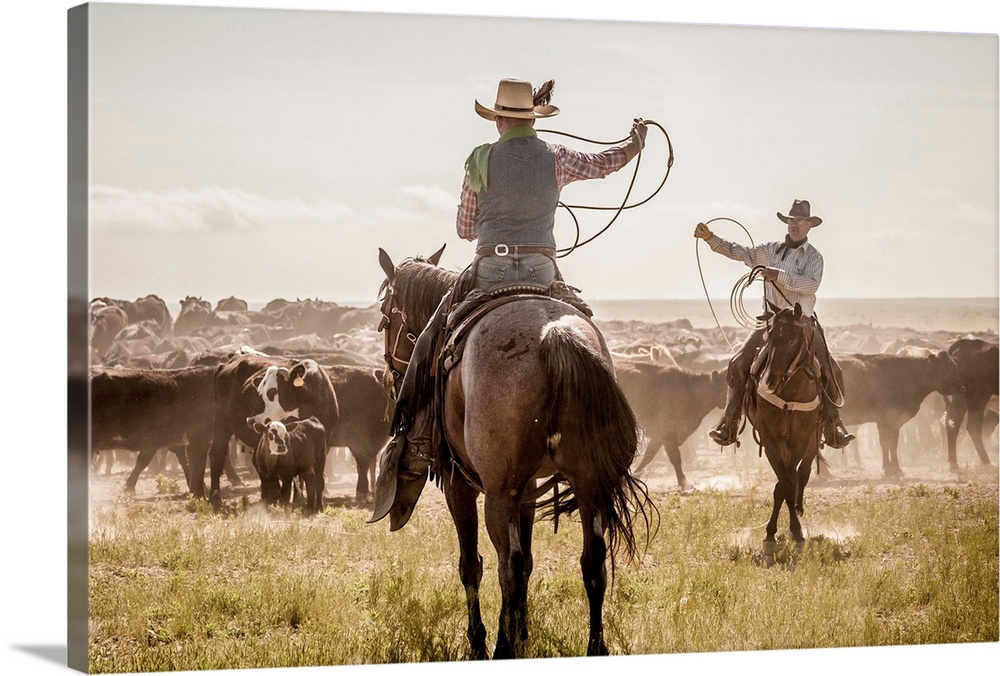The image depicts a dynamic scene of two cowboys on horseback at work, portrayed in a style suggestive of canvas artwork. Against a backdrop of a vast, dusty landscape under grayish skies with sporadic white clouds, the cowboys are poised to lasso a herd of cattle that stretches into the horizon. Tall, brownish-green grass surrounds them, adding texture to the scene.

The cowboy closest to the camera, riding a brown horse with dark legs and mane, wears a distinctive outfit comprising a red and white plaid shirt, blue vest, green scarf, denim jeans, brown cowboy belt, and a white hat adorned with a large feather. The second cowboy, facing the herd with his back to us, also sits astride a brown horse and dons a tan cowboy hat, a black scarf, a white shirt, and gloves suitable for roping. Both cowboys hold coiled ropes, ready for action.

The cattle in the background, some with ear tags, exhibit dark brown fur with white patches on their faces, indicating a mix of cows and calves. The rocky terrain visible in the distance, combined with the tall grass and the cowboys' detailed, traditional attire, immerses the viewer in an authentic Western wrangling scene.